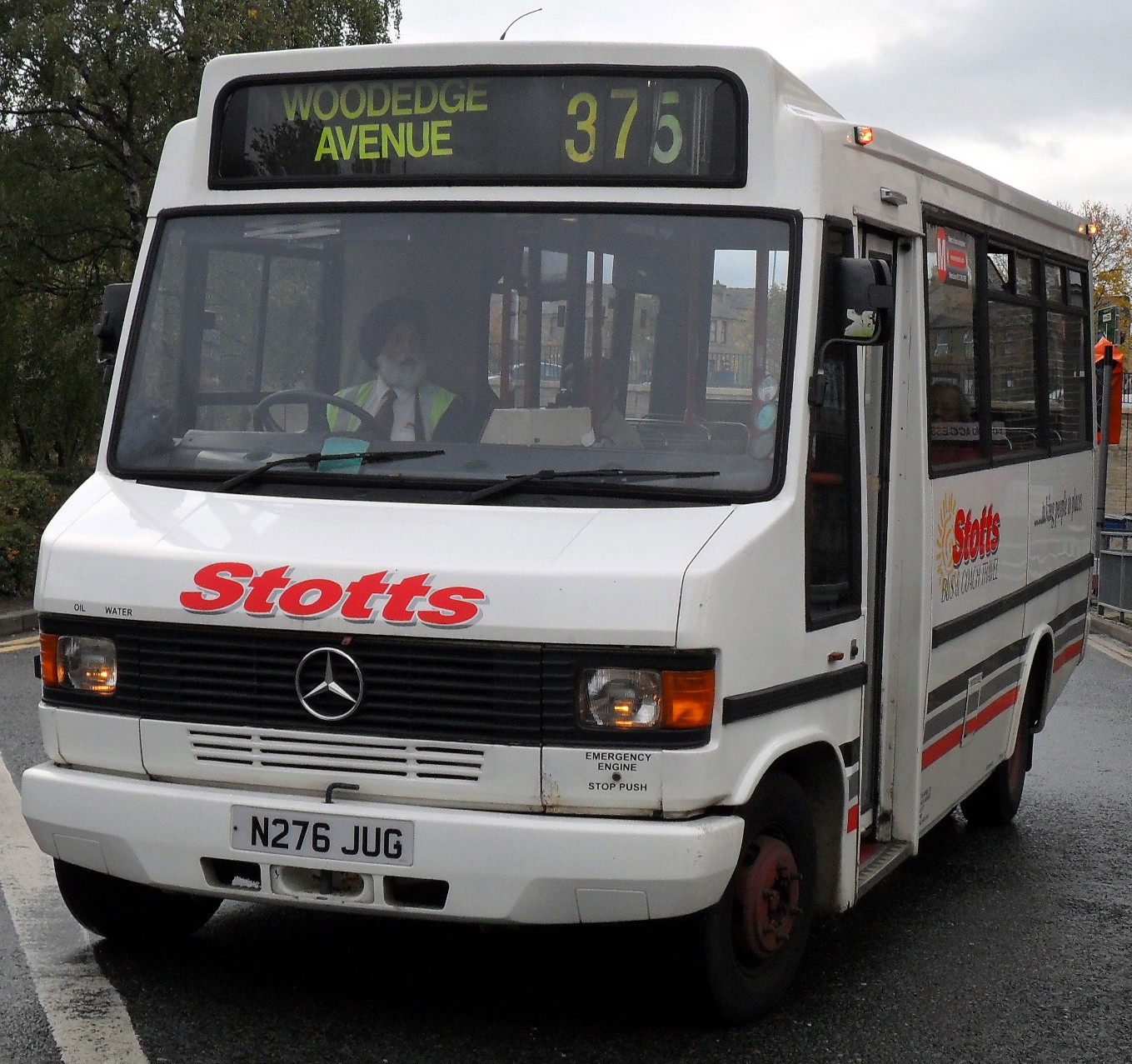This square outdoor photograph features a compact city bus, predominantly white with gray, red, and dark gray decorative trims. The bus, bearing the registration N276JUG, is viewed from the front and the passenger side, parked on an asphalt driveway. The bus is slightly larger than a typical shuttle but smaller than a conventional city bus, showcasing three windows along each side. Prominently displayed in red letters on the front grill is "STOTTS," along with the Mercedes-Benz emblem. Above the windshield, the bus's marquee reads "Woodedge Avenue 375" in a bright yellowish-green color.

Inside the bus, an older Indian male driver with a full white beard, dark turban, green jacket, safety vest, white shirt, and tie is visible. He is seated on the right side of the bus and seems to be looking off to the right. No passengers are visible inside the bus. The background features green-leaved trees and an overcast, gray sky, contributing to the overall serene yet functional scene.